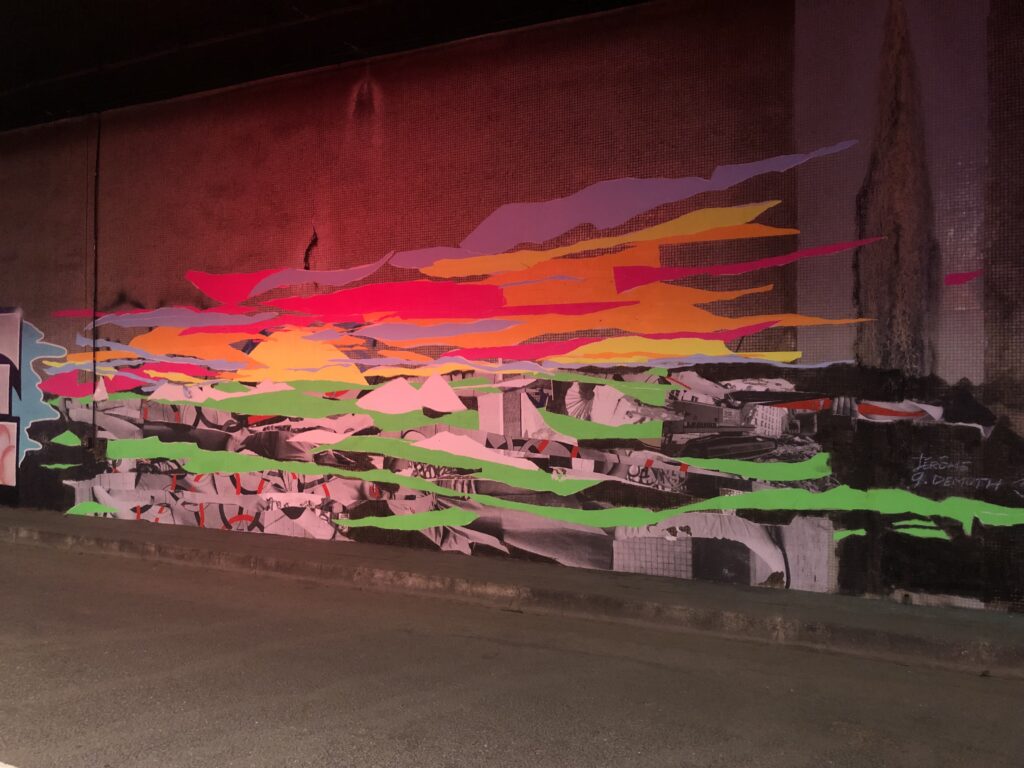This image captures a vividly painted wall along the side of a road, focusing on the intricate graffiti that adorns its surface. The top portion of the wall is unmarked, maintaining a bare, light gray color. As your eyes travel downward, the art becomes alive with a burst of colors and abstract patterns. Starting from the upper part, the artwork includes horizontal waves of red fading into purple, followed by a transition from purple to orange to pink. Below this, stripes of orange blend into yellow, red, and yellow again. The most prominent section features bright, fluorescent lime-green stripes that dominate the middle to the bottom of the wall. Interspersed within these green streaks are intricate black and white drawings, which appear to depict urban landscapes, including buildings and perhaps a sun. These black and white elements add a layer of complexity, contrasting the vibrant stripes that flood the wall. The entire composition suggests a chaotic yet visually engaging piece, possibly a spontaneous act of graffiti rather than a planned mural. Beneath the wall, a plain gray concrete road completes the scene, providing a stark contrast to the colorful explosion above.